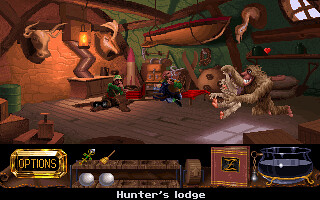This is a pixelated video game screenshot depicting a scene inside a rustic, cluttered lodge. The screen is dominated by earthy brown tones and features a green back wall. The room has wooden walls and floors, some planks appearing loose with gaps between them. At the bottom of the screen, the words "Hunter's Lodge" are printed in white letters on a black trim. 

In the lower left-hand corner, the word "Options" is displayed in bright yellow. Just below it sit two white balls on brown shelves. To the right, there is a gray cauldron with gold-colored feet, accompanied by a red book with gold trim and a gold letter 'Z' on its cover. 

The right side of the screen shows a light brown creature with big teeth, possibly a gorilla, leaping in the air amidst an assortment of household items, such as a boat hanging up, an ostrich head mounted on the wall, and various wooden objects like skis. 

On the left side, two characters dressed in green sit on the wooden floor, appearing to be hiding. The red brick wall with a stove and a pipe adds to the rustic ambiance, while lanterns and mounted animal heads contribute to the lodge's decor.